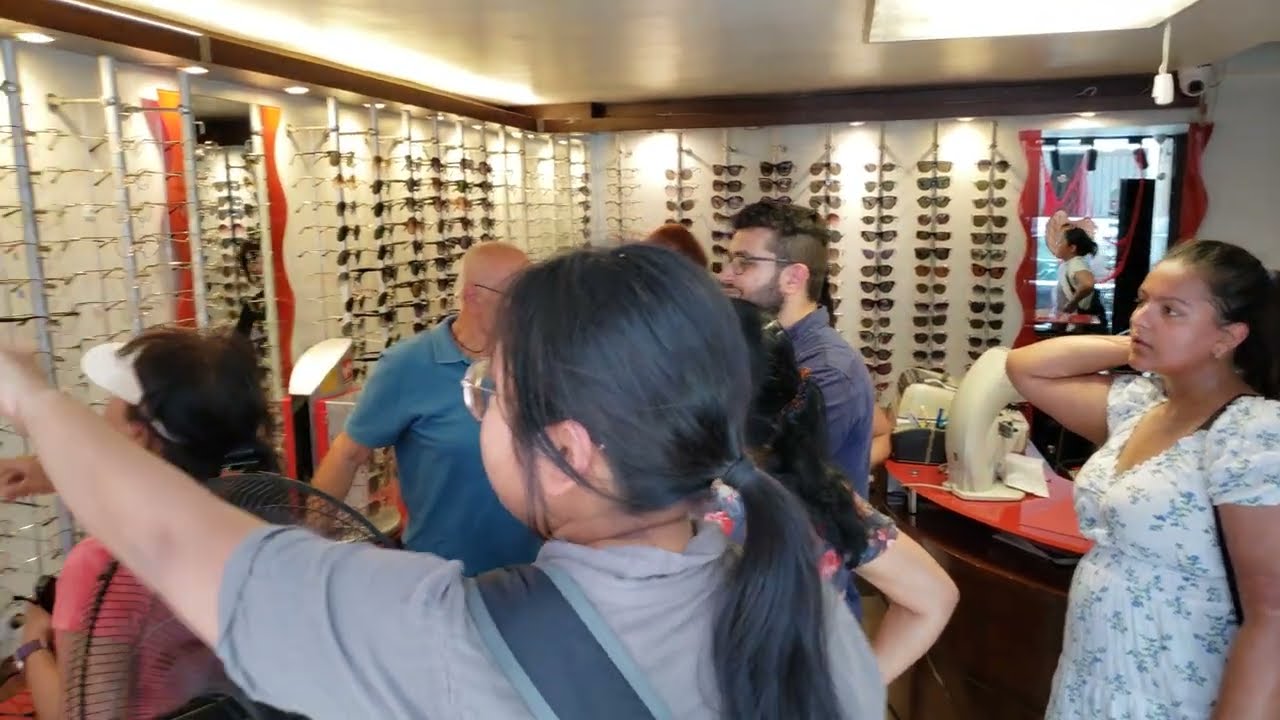The image depicts the interior of an eyeglasses store with a few individuals inside, roughly six people if one accounts for a visible reflection. The store features walls lined with shelves holding various eyeglasses, set at a 90-degree angle to each other, with a central mirror on the far left wall. There is a round, curved desk equipped with some machines on the right side of the image.

In the foreground, a woman with her long hair pulled back into a ponytail, wearing round glasses and a short sleeve gray shirt with a gray strap or bag over her shoulder, stands on the left side. She is pointing with her left arm raised toward the eyeglasses on the wall. To her right, a woman in a white short sleeve dress with a purse slung over her left shoulder and black hair partially obscured by the previous woman, stands next to a man facing the same wall. He is slightly angled and appears to be of Asian or Indian descent, wearing glasses. 

Adjacent to them, another woman with a visor and a pink shirt looks at the glasses, while a bald older man in a blue short sleeve shirt stands in the background. All individuals in the room appear to be intently focused on the array of eyeglasses displayed on the walls.